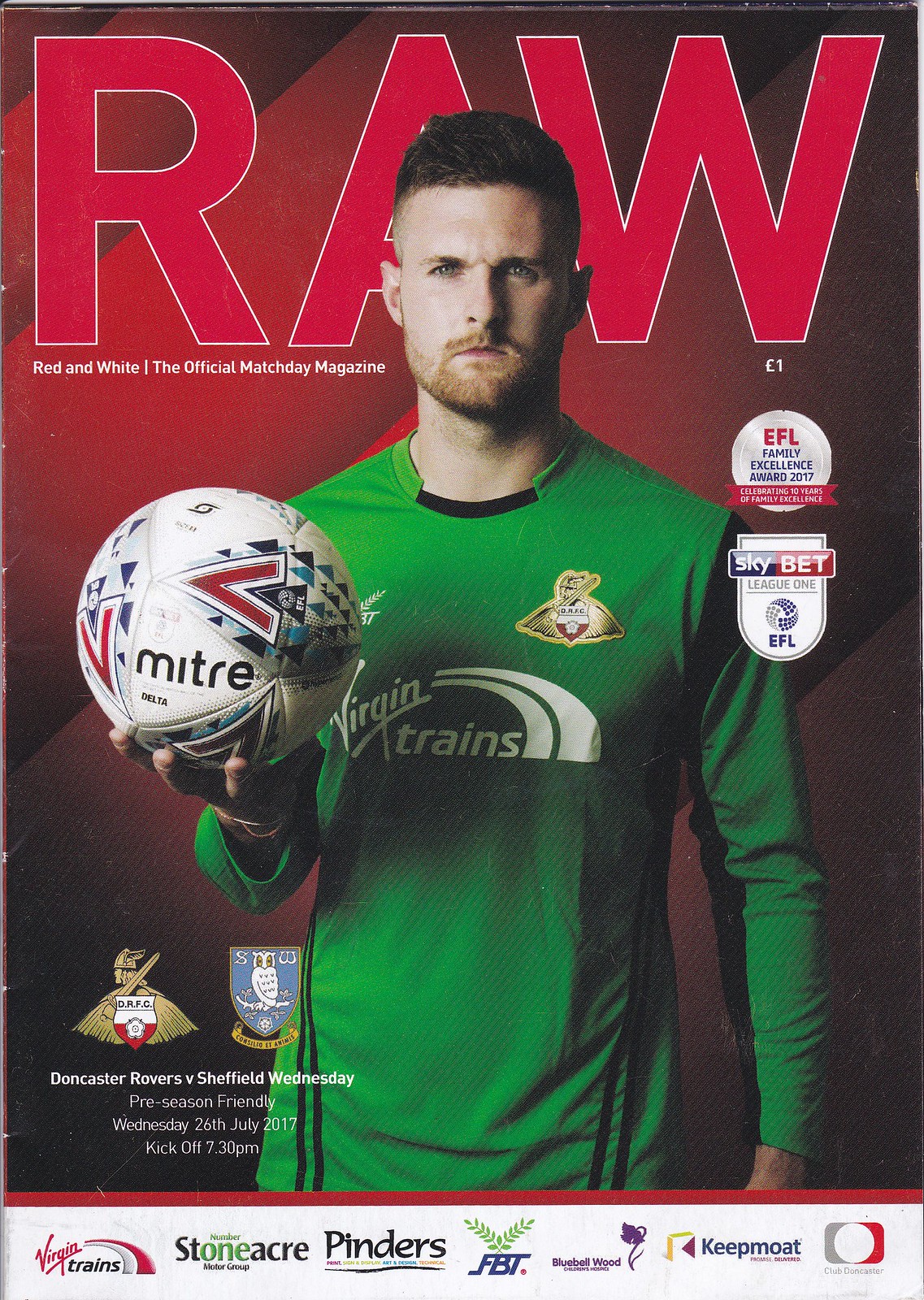This detailed magazine cover, titled "RAW," the official Match Day magazine for the Doncaster Rovers soccer club, prominently features a stern-faced man in a green jersey emblazoned with the Virgin Trains logo. He holds a soccer ball at chest level in his right hand. The top of the cover showcases the magazine's name in bold red font, with the subtitle, "Red and White, the official Match Game, Match Day magazine." To the center-right, two emblems are stacked: the top one reads "EFL Family Excellence Award 2017," and the one below says "Sky Bet League One EFL." In the lower left corner, there are emblems for Doncaster Rovers and Sheffield Wednesday, accompanied by text announcing a preseason friendly match between the two teams on Wednesday, 26 July 2017, with a kickoff time of 7:30 p.m. Bordering the lower part of the magazine are various sponsor logos, including Virgin Trains, Stoneacre Group, Pinders, FBT, Michael Wood, Keith Moat, and an illegible logo possibly related to the club.